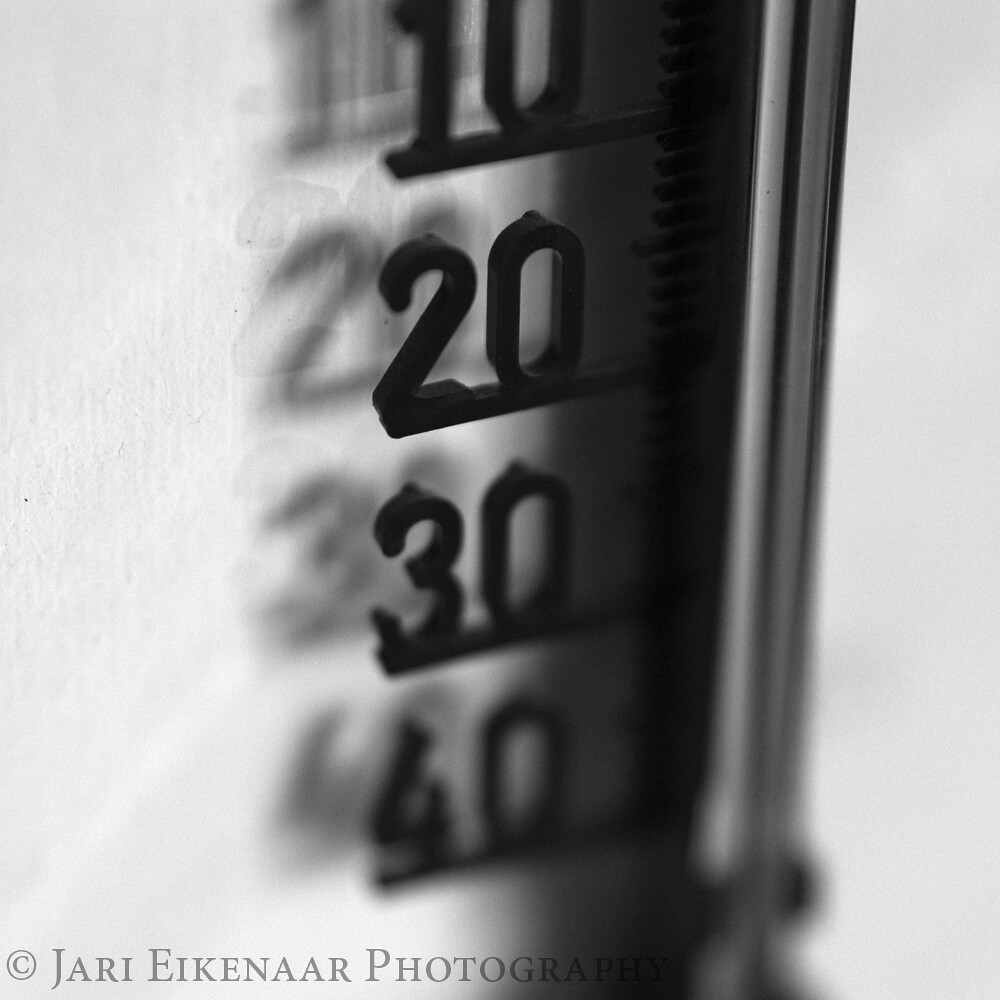In this captivating photograph by the legendary Jari Enkenar, located in the bottom left-hand corner, we observe a meticulous watermarked print of his work. The image itself is set against a pristine white background and prominently features a silver measuring instrument. The measurer, with its distinctive black comb-like notches and glossy, black, plasticky numbers, marks increments of 10, 20, 30, and 40. These numbers cast faint, intriguing reflections on the backdrop, adding depth to the composition. The photograph transitions into a beautiful blur towards the bottom, with the '40' slightly out of focus, demonstrating Enkenar's signature touch.